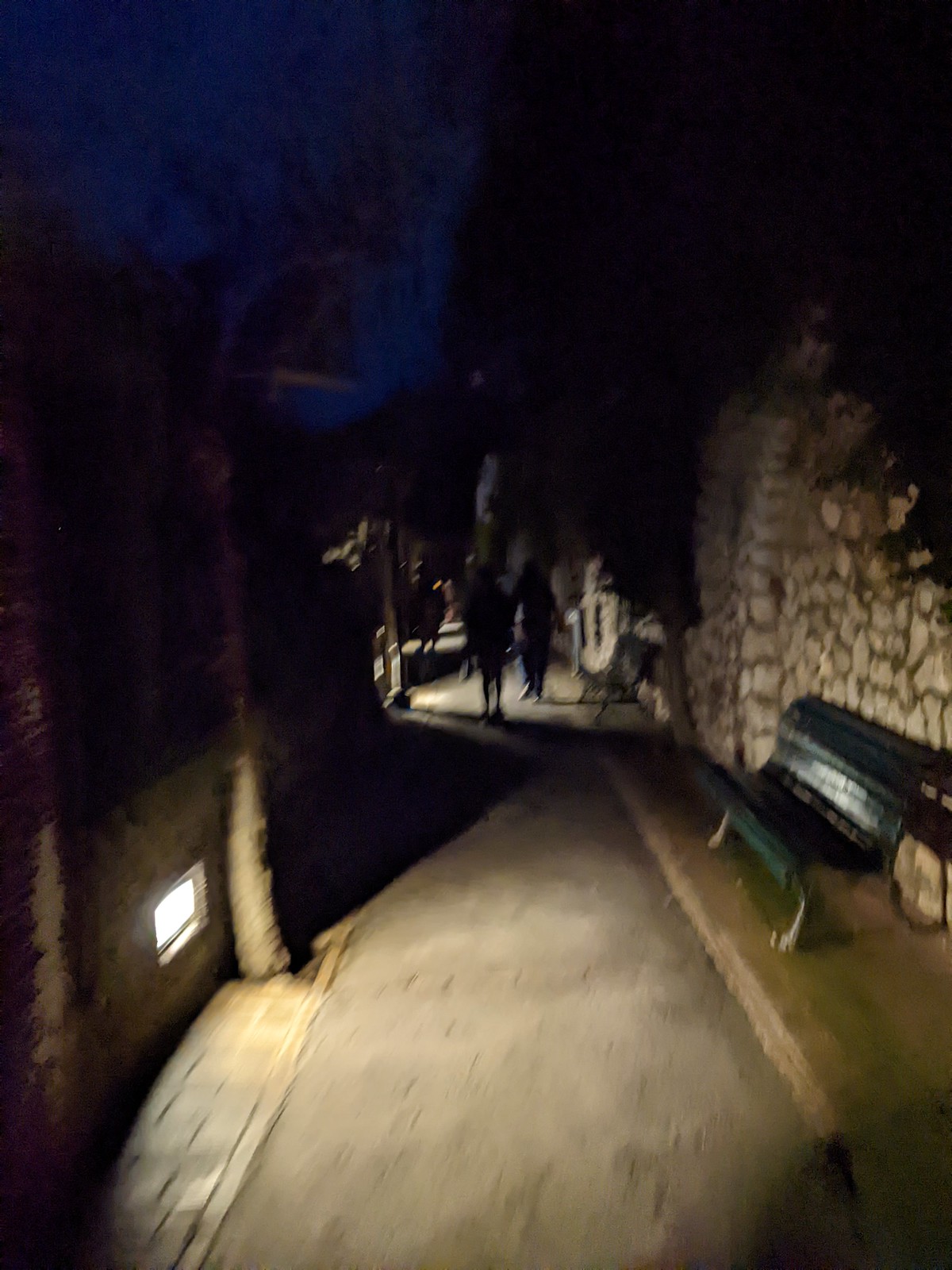A nighttime photograph reveals an enchanting walkway, dimly lit by a softly glowing light embedded within a nearby wall. The pathway, a mix of dirt and paving stones, is lined with brick pavers and a few trees rising from the ground. On the right side of the image, a green bench sits next to a curb, offering a quiet resting spot. Further down the path, shadows create a mysterious atmosphere, while the silhouettes of people are faintly visible in the distance. Vegetation cascades over the top of the wall, adding a touch of nature to the scene. Despite the darkness, the light provides just enough illumination to reveal the intricate details and serene ambiance of the setting.